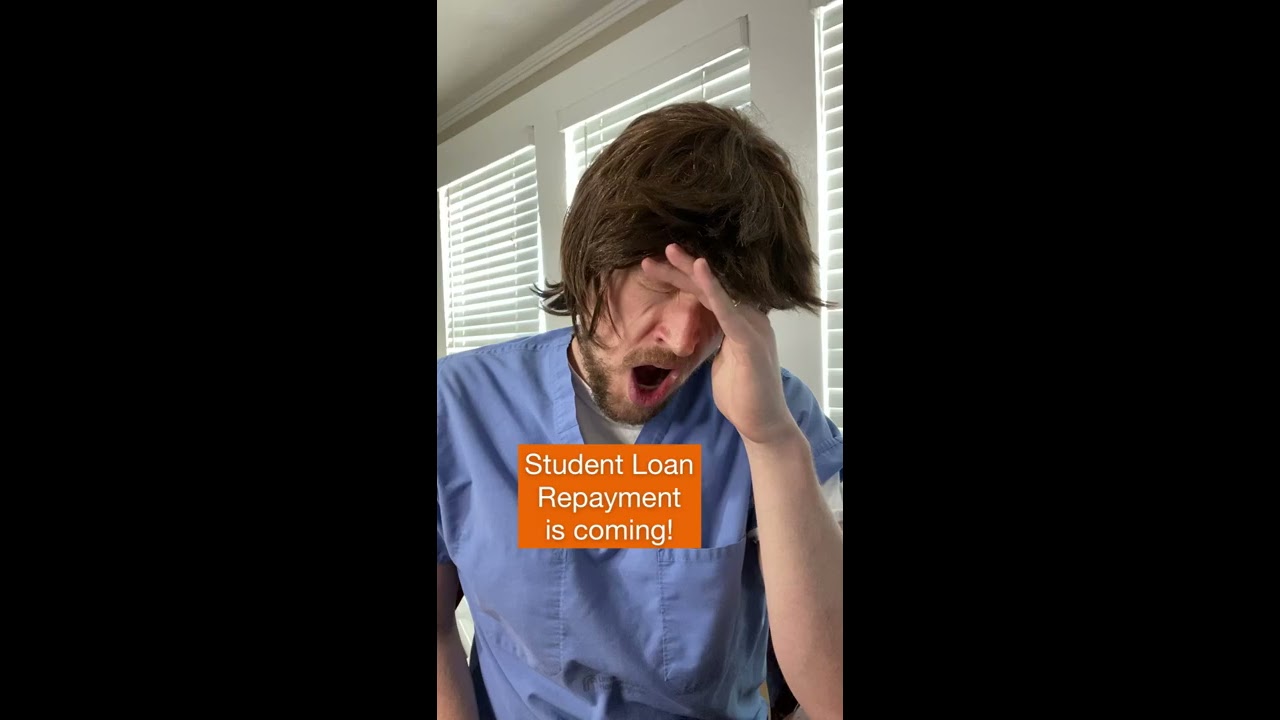In the image, there is a man, likely a medical student or nurse, captured mid-yawn or expressing frustration, wearing muted blue scrubs with a white t-shirt underneath showing through the V-neck. His messy, long brunette hair is partially covering his eyes, held back by his left hand positioned on his forehead. His right hand rests at his side, revealing a gold ring. The man's expression is one of apparent tiredness or worry, likely about the impending "student loan repayment," as indicated by the orange rectangle with white text near the bottom of the image. Behind him, the setting includes white blinds partially covering three windows, edged with white wooden borders, and a white ceiling above. The image is framed with wide black bars on the left and right, suggesting that this is a screenshot from a portrait-oriented video, possibly shared on social media. The colors present in the image include various shades of blue, white, brown, peach, and gold, highlighting the visual elements and contributing to the overall somber mood.